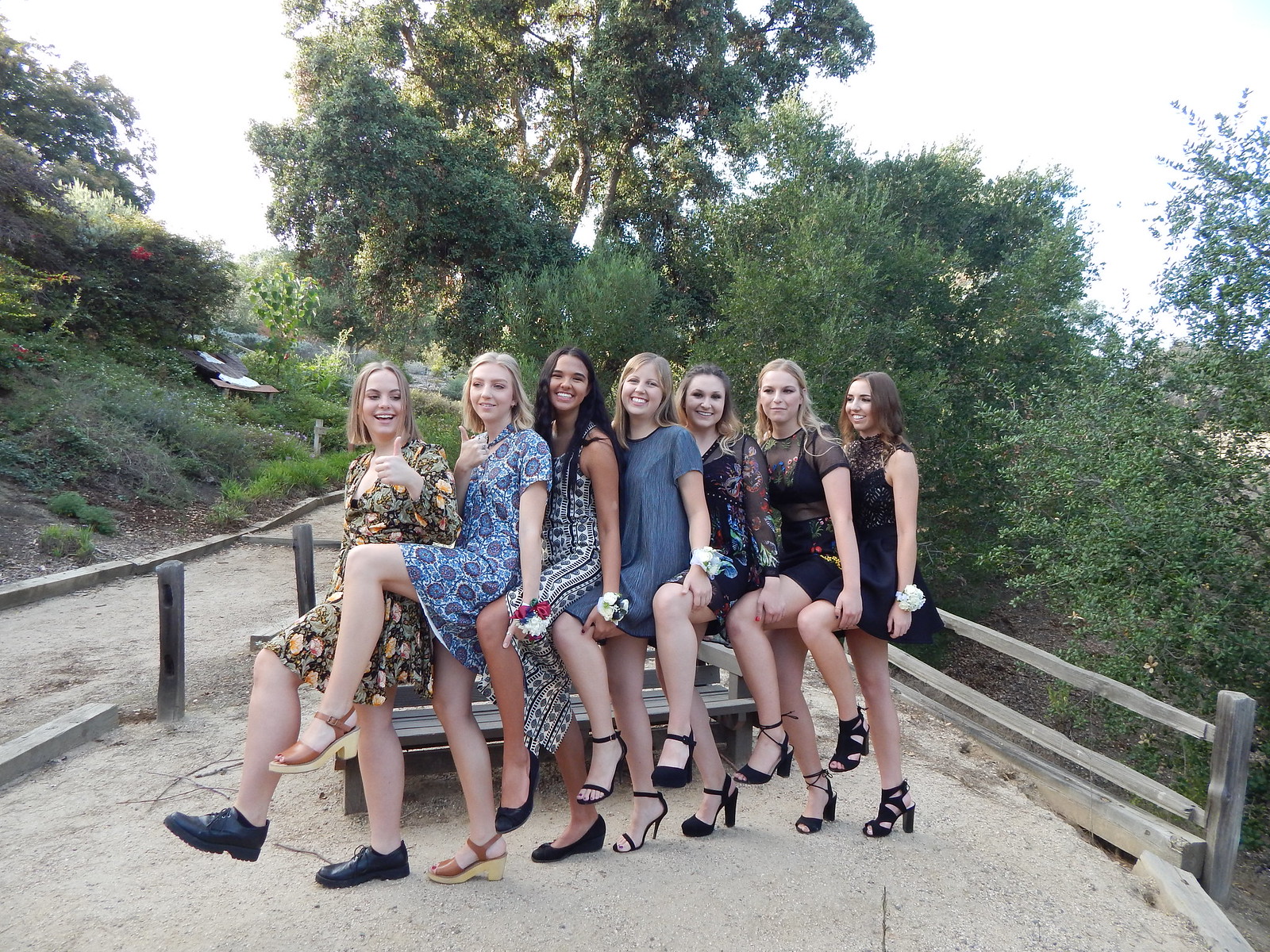In the image, seven young women, possibly in their late teens or early 20s, are posing in a line on a gravelly path surrounded by lush greenery and trees. The setting appears to be a scenic hiking trail or wooded area, with a stockade fence on the right and a wooden barrier on the left. Each of the women is standing with her left leg raised, knee at hip height, while the right leg is bent to the ground. They are all looking at the camera and smiling, exuding happiness. The women have short hair and are dressed in various eye-catching outfits, including green and blue floral dresses, an all-blue shirt dress, and a black dress accented with a white flower on the arm. Some are wearing black heels while others have more sturdy shoes, and four of the women wear corsages on their left wrist. The background features a garden of greenery with hills and trees, adding to the serene outdoor ambiance.